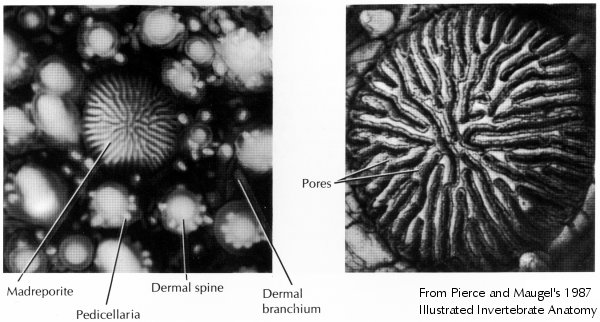This image features a detailed black-and-white diagram presented in a side-by-side format. The first section of the diagram is zoomed in on skin-like structures and is intricately labeled. The prominent center cell is labeled as "Madreporite," surrounded by smaller white circles identified as "Pedicellaria," along with additional labels pointing to the "Dermal Spine" and "Dermal Branchium." 

The adjacent section provides an even closer view of the "Madreporite," highlighting the texture and intricacies with numerous squiggly lines, each marked as "Pores." At the bottom of the second image, there is a reference to the source: "From Pearson Magel's 1987 Illustrated Invertebrate Anatomy," suggesting this diagram is an educational illustration focusing on the anatomy of invertebrates, specifically detailing skin cells and pore structures.